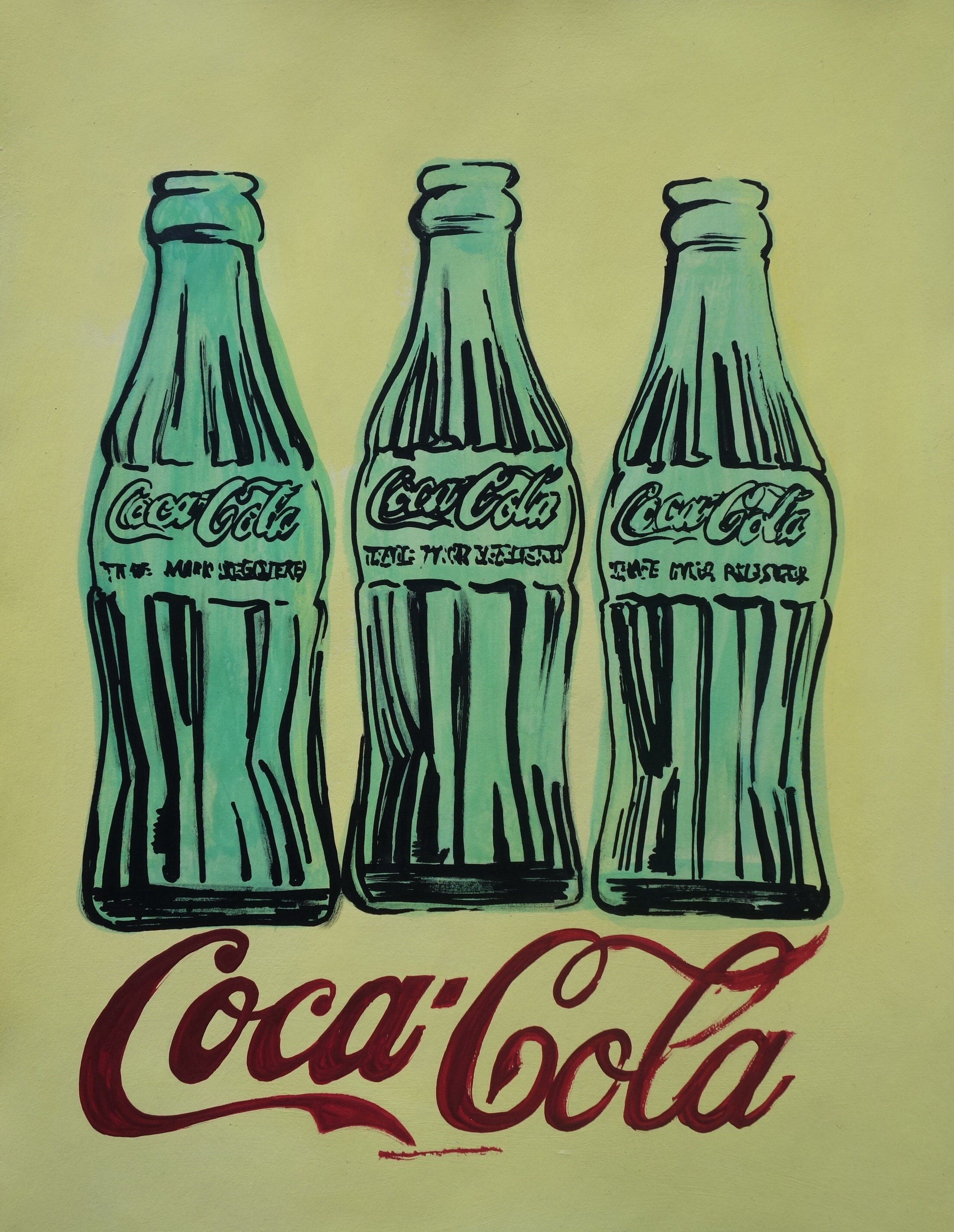This is a color drawing on a light yellow background featuring three iconic, old-time Coca-Cola glass bottles. The bottles are artistically rendered, tinted blue with vertical black lines that add texture. Each bottle has the classic Coca-Cola shape: wide at the bottom, narrowing upward, then bulging outward before tapering to the top. They are depicted without caps and appear empty. 

Centered on the front of each bottle, the Coca-Cola logo is displayed in a bold, red cursive script. Below the logo, there is some additional text that remains unreadable due to its unclear rendering. A similar red Coca-Cola logo is repeated at the bottom of the image, above a thin red line. The bottles are spaced evenly side-by-side and reveal an abstract artistic touch with green paint streaks that sometimes extend beyond their outlines. 

The overall style combines elements of a sketch and a painting, complete with hand-painted aspects that give an impressionistic, slightly messy appeal, adding to its vintage advertisement vibe.